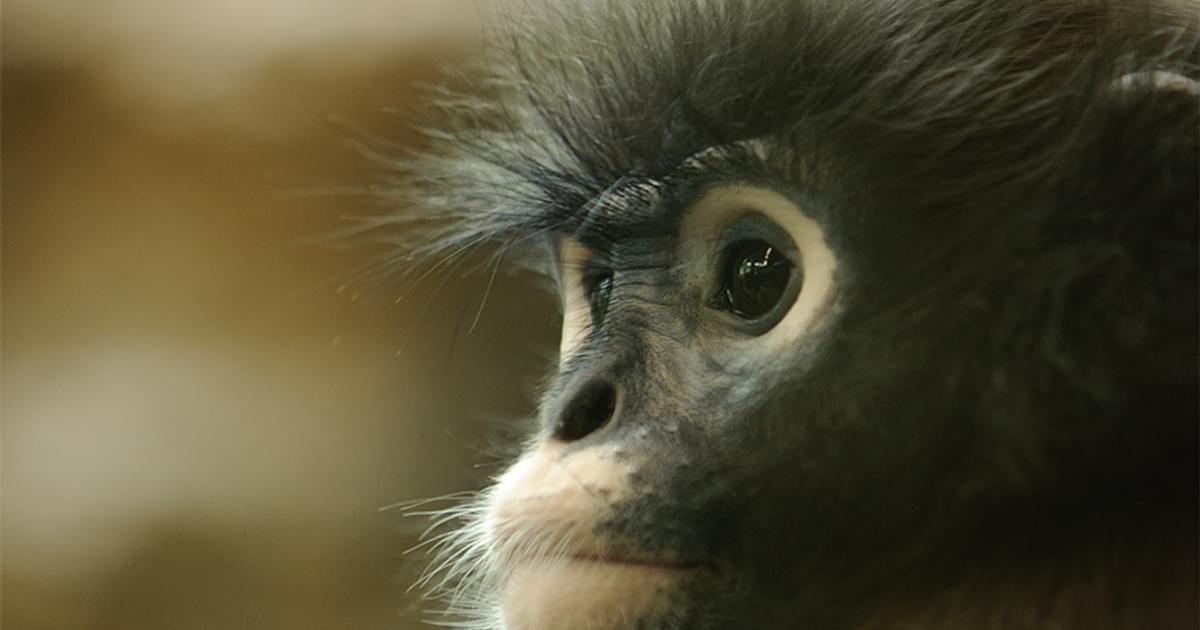This close-up photograph captures the side profile of a young monkey, possibly a baby, occupying the entire right side of the frame. Its face is small and predominantly black, with striking features that include dark, black eyes encircled by white or whitish pink rings, and a tiny, white-lined mouth adorned with white whiskers. The monkey’s black nose stands out against its black fur, which appears soft and fluffy, adding to its juvenile look. Only part of one ear is visible in the upper right corner of the image. The background, occupying the left side, is entirely blurred with a mix of brown, tan, and white hues, hinting at a natural setting. The monkey is looking away from the camera, perhaps slightly forward, contributing to an enigmatic and serene composition. The focus on the monkey's detailed features against the blurred background enhances its prominence and the texture of its fur.